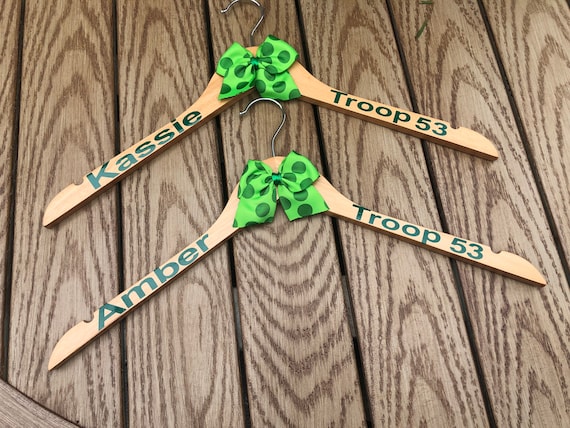Resting on a vertically aligned wooden surface, there are two wide wooden hangers adorned with silver hooks. Each hanger features a vibrant, fluorescent green bow adorned with dark green polka dots. The top hanger bears the name "KASSIE" in Kelly green print, followed by "Troop 53." Similarly, the hanger below is labeled "Amber" and also references "Troop 53," both in the same stylish Kelly green font. The overall presentation is neat and colorful, adding a personalized touch to the wooden hangers.